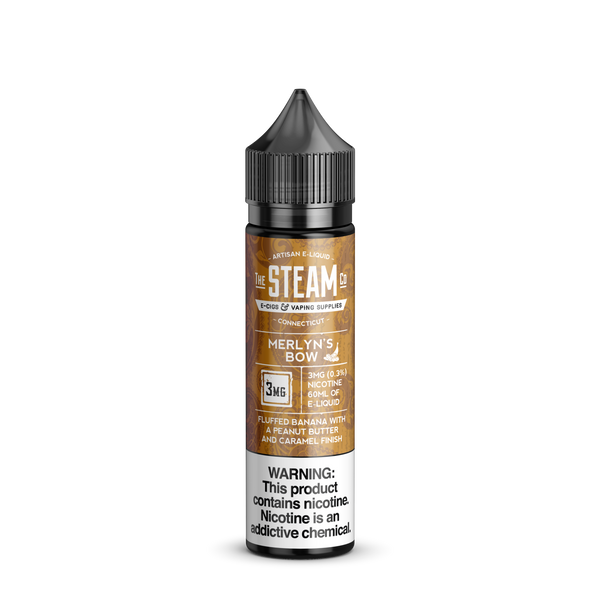The image features a tall, cylindrical bottle with a black, pointed twist-off cap featuring grooves for an easy grip. The bottle stands against a completely white background, commonly seen in retail images or promotional photographs. The midsection of the bottle has a distinct, burlwood-colored label with various texts. At the top of the label, it states, "Artisan E-Liquid Steam, E-Cigs, and Vaping Supplies, Connecticut," in white text. Below this, there is a white line followed by the product name "Merlin's Bough" next to a decal resembling a white bird. Further down, it details "3MG, 0.3% nicotine, 60MHL of E-Liquid," and describes the flavor as "Fluffed Banana with a peanut butter and caramel finish." The bottom 25% of the bottle is a white section with black text prominently warning, "This product contains nicotine. Nicotine is an addictive chemical." The entire setup appears to be designed for clear, informative display typical on retail websites.